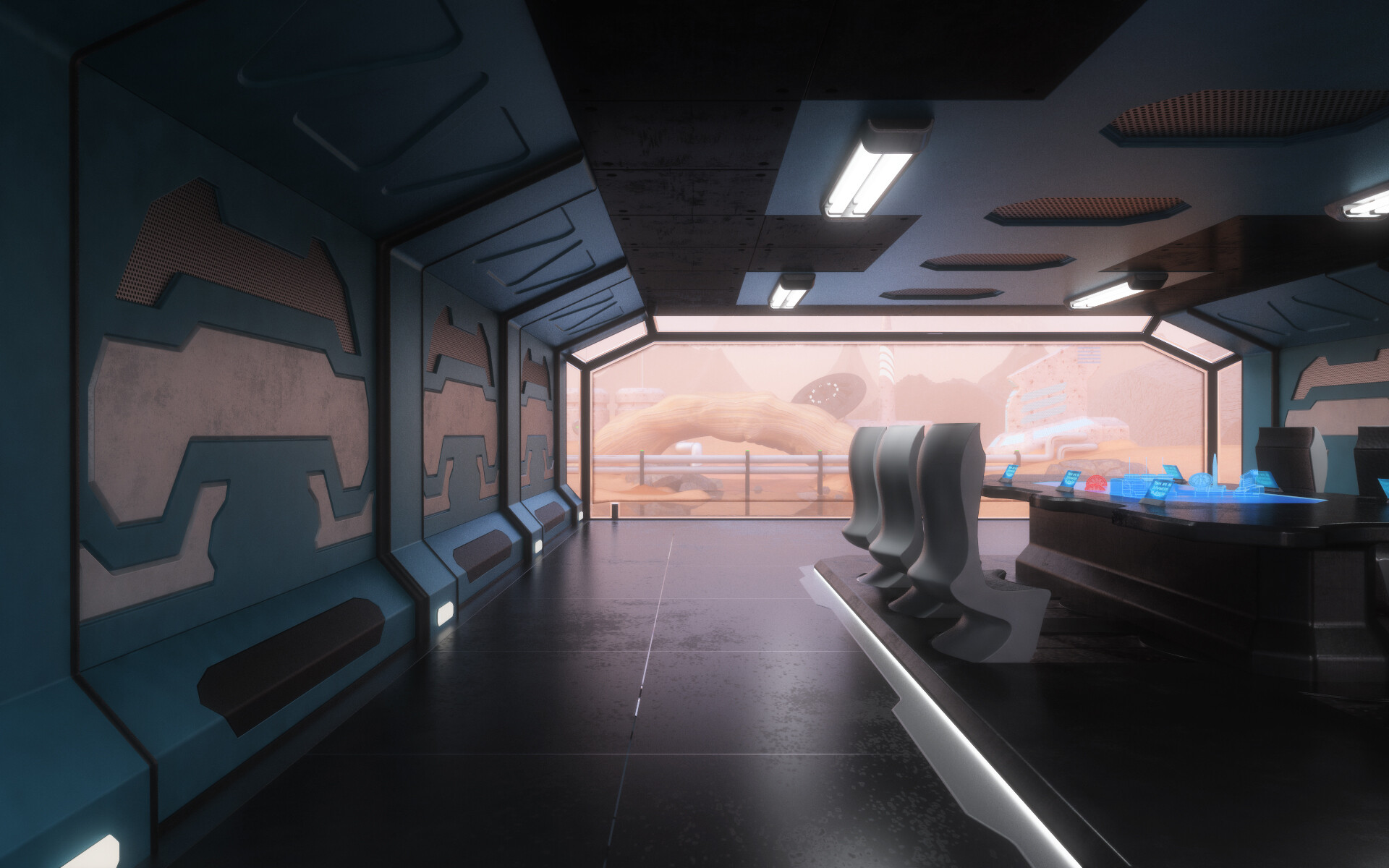This color photograph captures a highly detailed, futuristic conference room, evoking a sci-fi atmosphere reminiscent of a spaceship or an advanced control center. Dominating the room is a sleek, black conference table flanked by ergonomically designed, sculptural white chairs. Each seating station is equipped with small, glowing tablet-like screens. Central to the table is a striking 3D hologram, emitting an icy blue light and possibly depicting a scene of futuristic buildings, adding a palpable air of technology.

The room is bathed in dim lighting, enhancing the modern ambiance, with the ceiling adorned with industrial dark gray and dark blue hues complemented by four long, fluorescent light panels. The walls, lined with grayish-blue colors and bearing a sandstone-like pattern, further accentuate the advanced design of the space. 

A distinctive feature is the vast window stretching across one end of the room. This window reveals an otherworldly, reddish-toned landscape filled with geometric, futuristic structures that hint at an extraterrestrial environment. A white fence and what appears to be a patio or platform are visible outside, adding depth to the scene. The black tiled floor and the sleek, black and brown patterned walls complete the room's ultra-modern aesthetic.